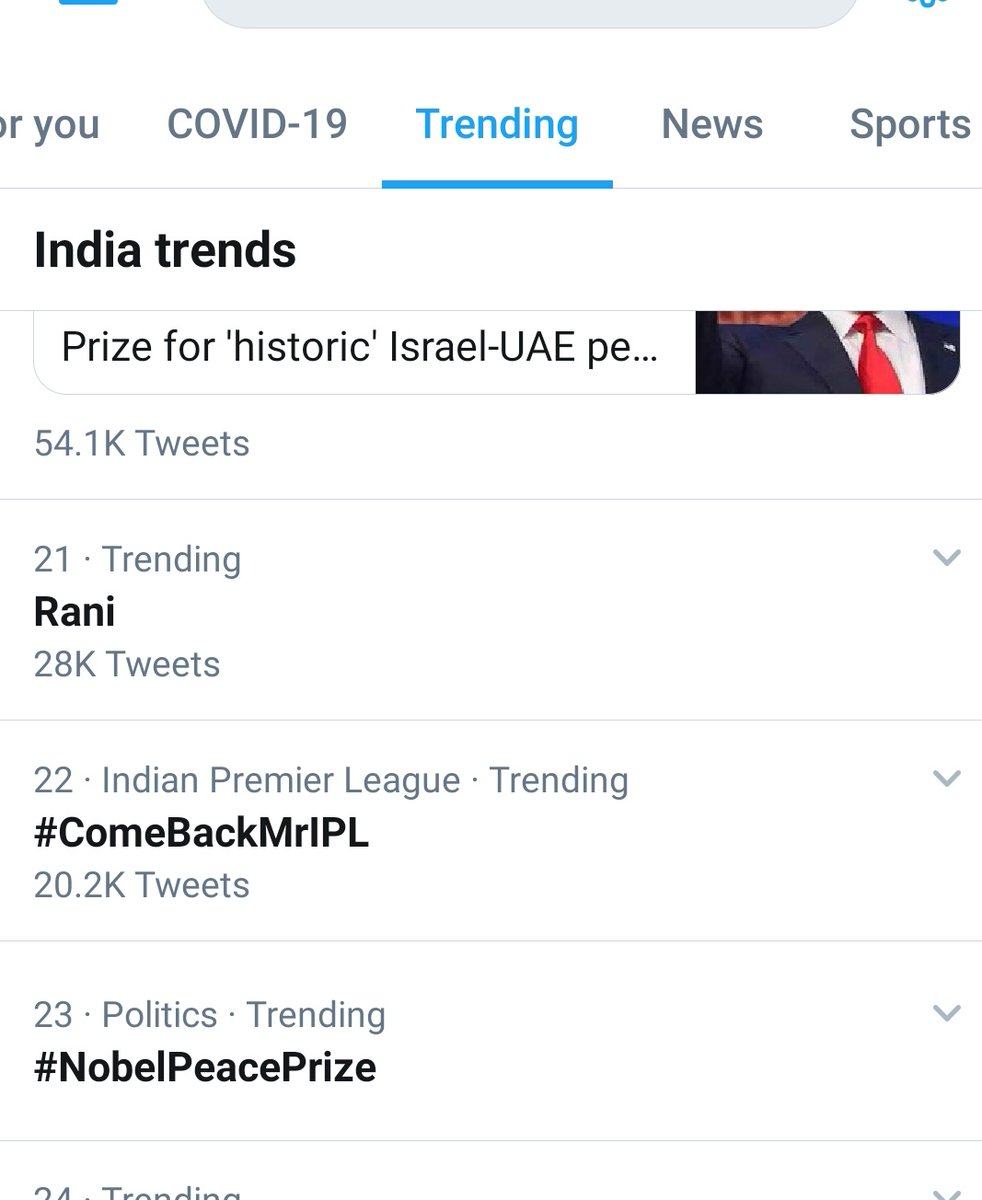This is a cropped screenshot of Twitter's trending section, displayed against a white background. There are several categories listed across the top of the screenshot: "For you," "COVID-19," "Trending," "News," and "Sports." The "Trending" category is highlighted in blue with corresponding blue text and an underline.

Below these categories, a vertical list of trending topics is visible. At the top, "India trends" is prominently displayed in bold black font. Directly underneath this, the trending article "Prize for Historical Israel UAE..." is listed, accompanied by a partially cut-off thumbnail image on the right.

Following this, the 21st trending topic is "Ronnie," also in bold black font, with the number of related tweets shown underneath. The 22nd and 23rd trending topics are also included. The 22nd trend is "Indian Premier League," with a subtext "#ComeBackMrIPL." The 23rd trend, categorized under "Politics," is "#NobelPeacePrize."

This detailed depiction captures the specific elements and hierarchical structure of the screenshot.